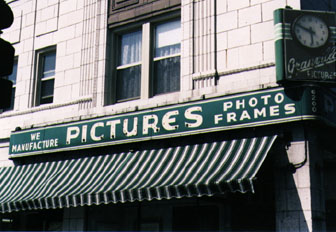This photograph captures the exterior of a vintage white brick building, reminiscent of structures from the 1920s to 1940s, situated in a bustling downtown area. Dominating the facade is a prominent green banner that reads "We Manufacture Pictures, Photo Frames," which suggests the building houses a photography or framing business. Complementing this banner is a striped awning in matching green and white hues, providing a cohesive aesthetic to the storefront.

At the top right-hand corner of the building, a metal clock is affixed, displaying the time as 5:50. The clock features a white face with green accents and some indistinct lettering, likely indicating the brand or name of the photo shop. Above the green banner, two windows enhance the building’s nostalgic charm. The overall scene creates an impression of a bygone era, steeped in historical character and urban vibrancy.